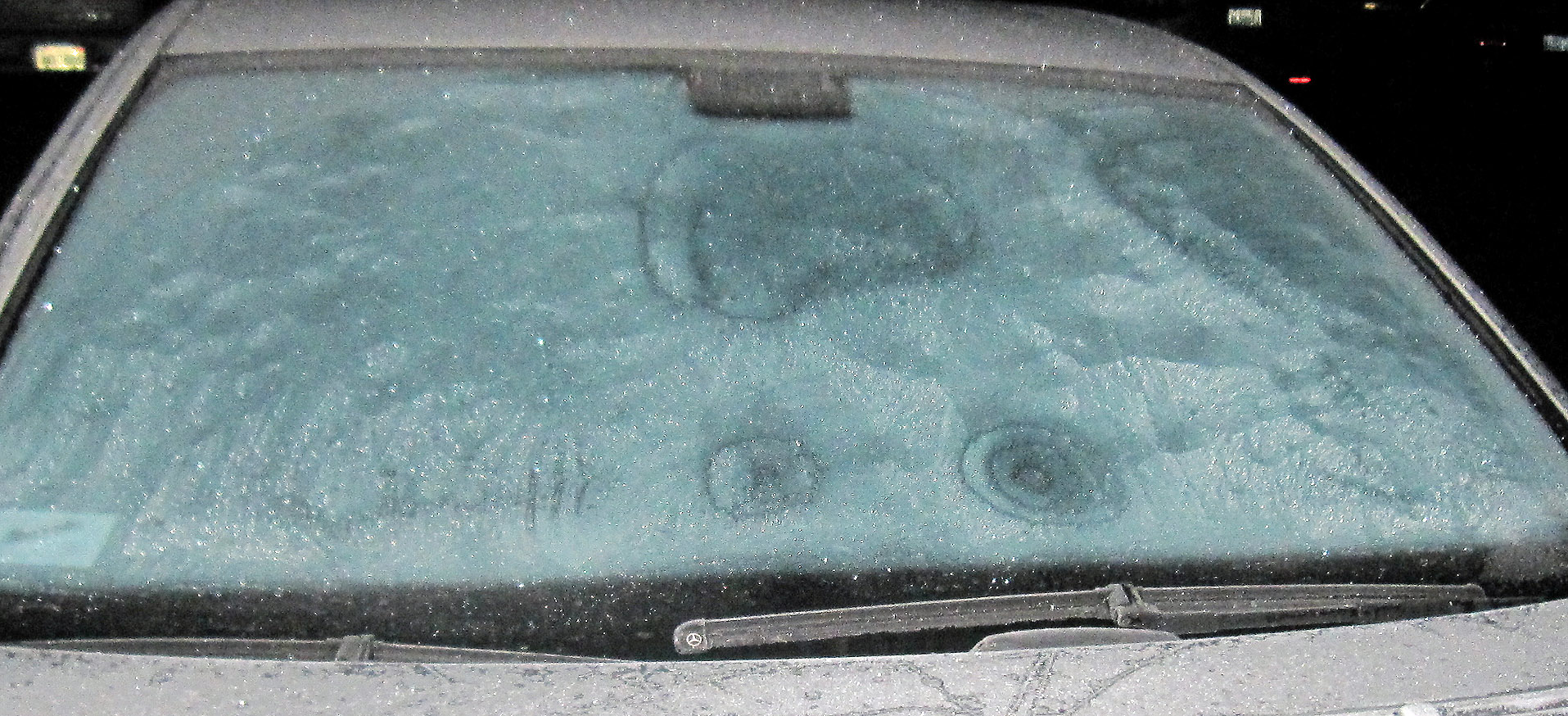The image captures a white car’s windshield enveloped in a light turquoise-green hue of frost and snow, set against a starkly dark background, enhancing the contrasting details. Photographed from the hood, it appears to continue snowing, evident from the myriad of white dots scattered across the windshield. Central on the windshield, an irregular, slightly rounded pattern emerges at the top, indicating an attempt to wipe the ice. Below this, near the center, is a smaller circular mark, as if drawn by a finger. To the right of this, a larger circular pattern encompasses two progressively smaller circles, creating a distinctive design amidst the frosted surface.